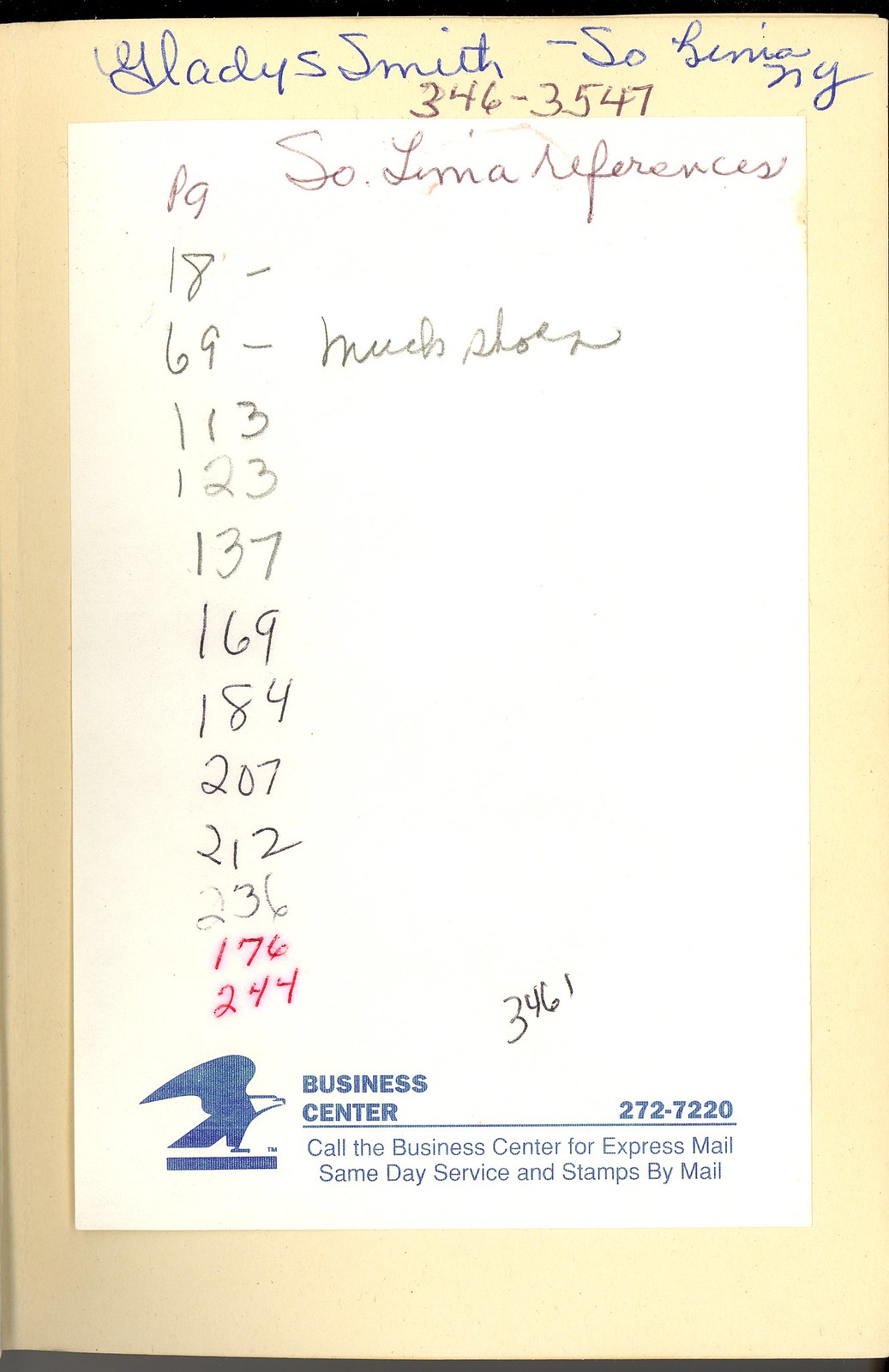The image depicts a light brown piece of paper with a white rectangular slip pasted in the middle. The white slip, which seems to originate from the U.S. Postal Service, features various handwritten notes and printed text. At the top, in blue ink, is written "Gladys Smith Soe Hiening." Below this, in brown ink, are the words "346-3547 Soe Lama references page 1869 113 123 137 169 184 207 212 136." Additionally, the numbers "176" and "244" are written in red ink. The lower part of the slip displays printed text in blue with an eagle logo to the left and the following message to the right: "Business Center 272-7220. Call the Business Center for express mail, same day service, and stamps by mail." The entire setup, bordered by a light pink frame, resembles a scrap paper or a business notebook sheet, possibly from a hotel.